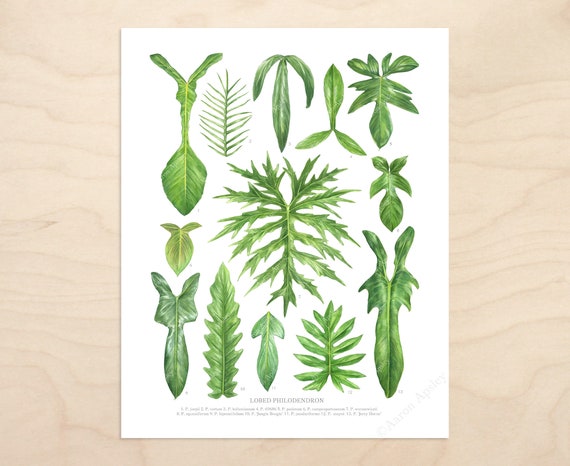The image showcases a detailed, scholastic illustration laid out on what appears to be a whitewashed wooden table. The illustration features approximately 13 green leaves resembling various plants, each meticulously drawn to highlight their unique shapes and shades of green. This scientific chart or poster, likely intended for use in a classroom or science lab, displays the plants' scientific names in Latin at the bottom, with legible black text that is easy to read. Each plant is numbered, suggesting that these correspond to additional information or descriptions. The bright and professional style of the illustration makes it an effective educational tool, emphasizing clarity and realism in the depiction of the plants' leaves.